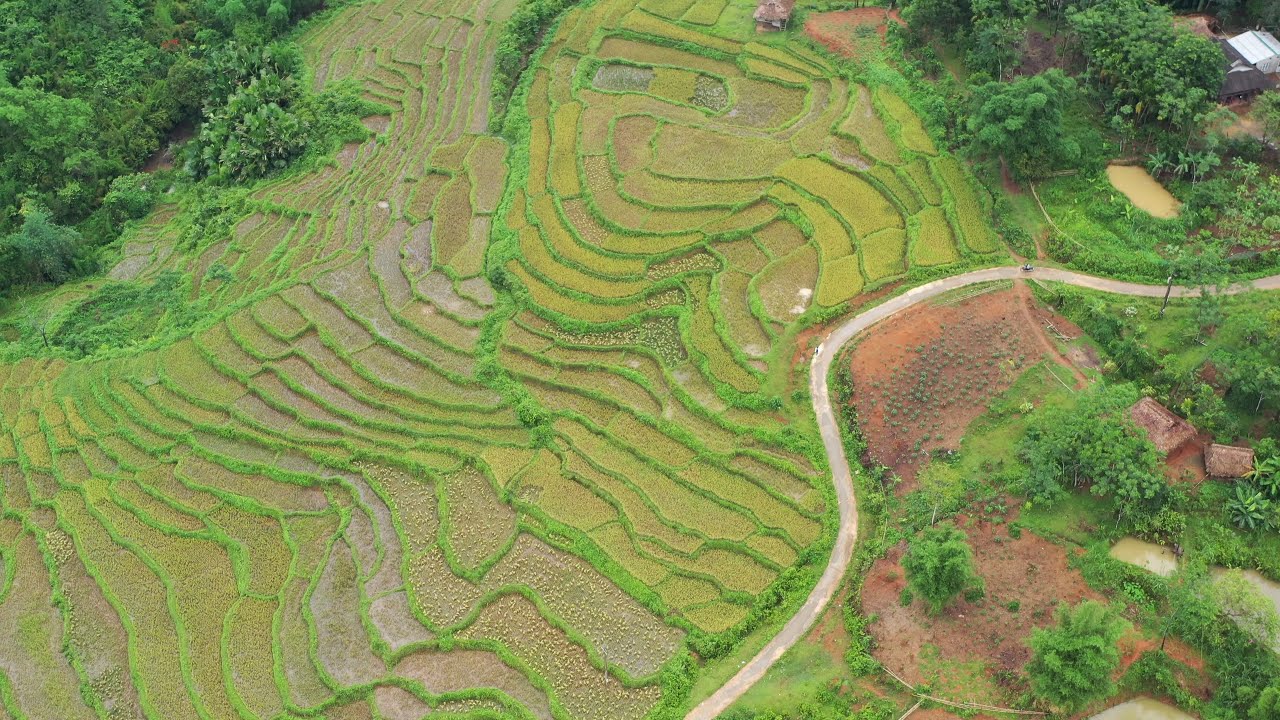This aerial photograph, likely taken by a drone, captures an expansive view of green fields and terraced farmland set in the countryside. The upper corners of the image are dense with bushes and trees, creating a natural frame for the scene. The central portion of the image showcases the terraced fields with distinct, wave-like patterns formed by bright green foliage that outlines various sections of land. These sections appear somewhat irregular in shape and are bordered by growth, suggesting preparations for potential flooding or irrigation. The fields feature alternating strips of grass, dirt, and new plant growth, contributing to a patchwork effect.

A small, winding, single-lane road cuts through the landscape, beginning at the bottom center and curving up to the right before disappearing off the edge of the image. The road is paralleled by scattered trees and a mix of rocky and bare patches of ground. In the bottom right corner, additional clusters of trees and bushes are present, adding to the rural charm. The upper right corner also includes a small building, possibly a house, beside a tiny brown pond, which hints at a habitation amidst the agricultural expanse. The overall scene evokes a sense of serene, cultivated land segmented by both natural and man-made boundaries.